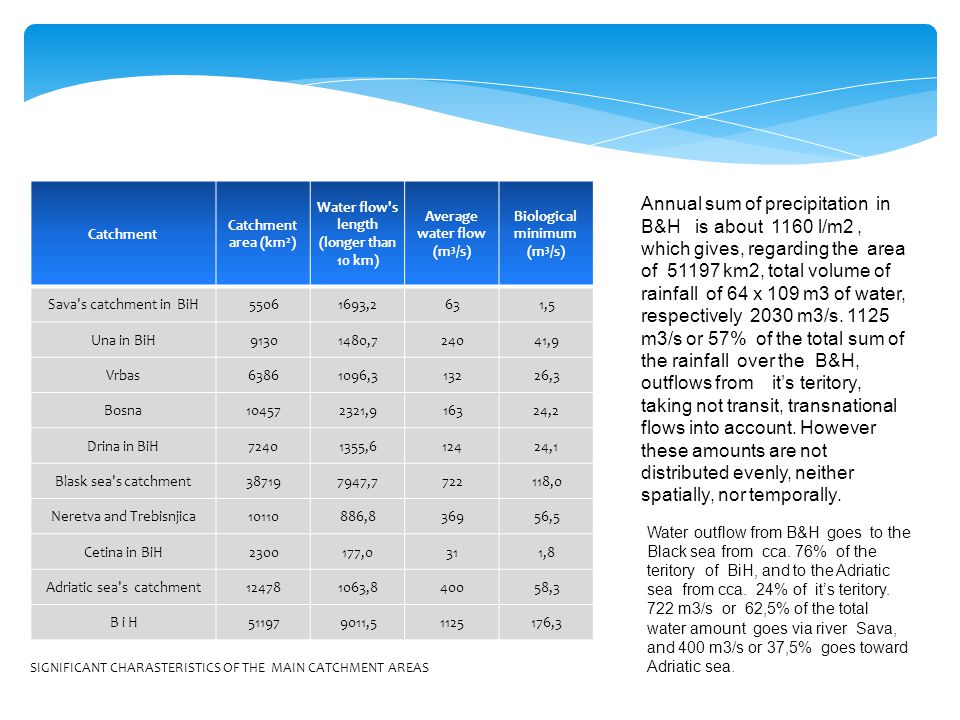The image appears to be a detailed page from a textbook, focusing on the hydrology of Bosnia and Herzegovina (B&H). The centerpiece is a graph that outlines key metrics related to water catchment areas. The graph, presented with white text on a blue background, showcases five categories: "Catchment," "Catchment Area in kilometers," "Water Flow Length Longer Than 10 kilometers," "Average Water Flow," and "Biological Minimum." Each category is populated with various numerical values. To the left of the graph, specific catchment areas such as Sava, Una, Vrbas, Bosna, and Derna are listed, indicating their flow towards different basins, including the Adriatic and Black Seas. The top of the graph includes a title mentioning "Significant Characteristics of the Main Catchment Areas," and a note on the bottom left echoes this focus. On the right side of the page, two paragraphs provide additional context, stating that the annual sum of precipitation in B&H is 1160 millimeters, covering an area of 51,000 square kilometers, contributing to a considerable total volume of rainfall. The text explains the uneven spatial and temporal distribution of this precipitation, noting that 62.5% of the total water volume flows via the River Sava, while the remaining 37.5% heads towards the Adriatic Sea. Aesthetically, the page is highlighted by a blue curvy design at the top.